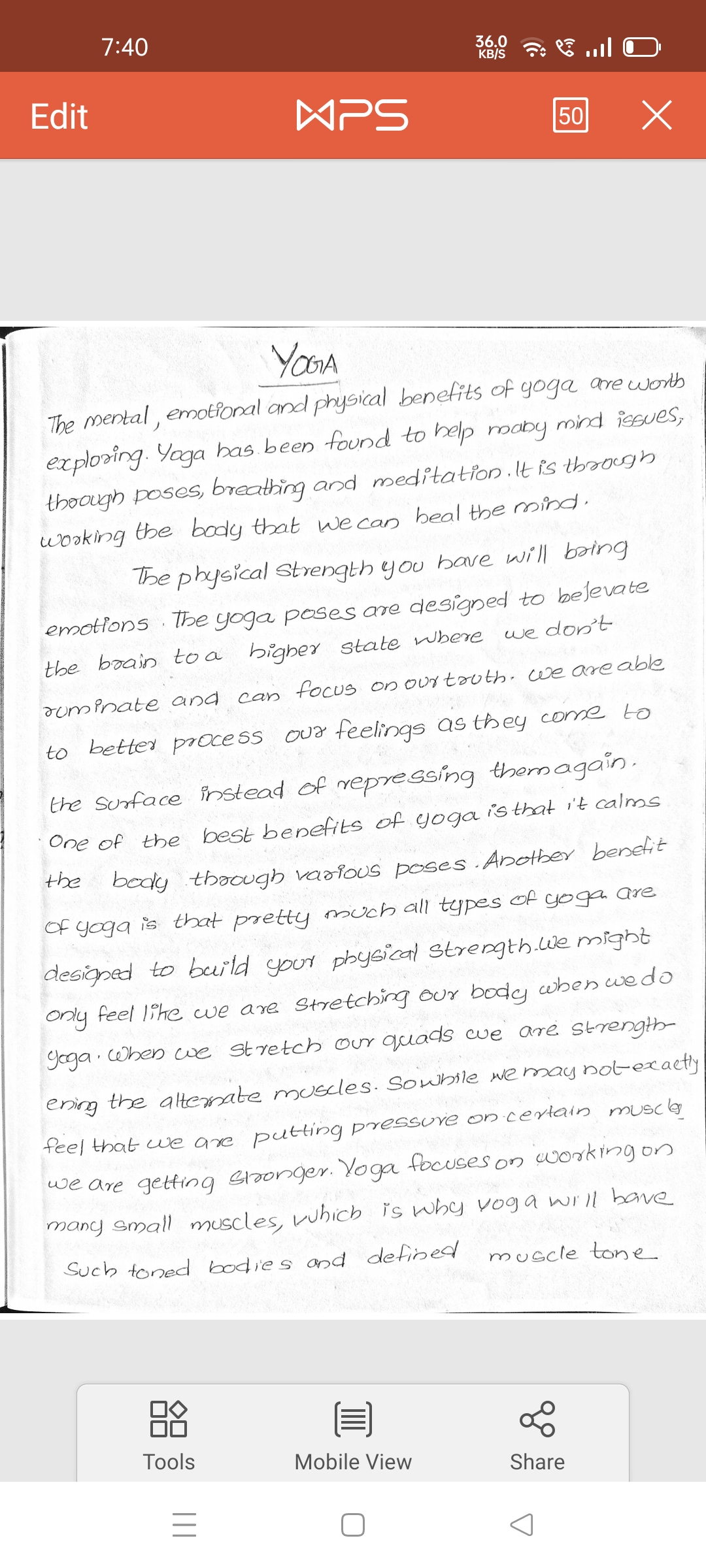The image captures a section of a device screen with the top portion shaded in maroon. The time displayed is 7:40, and the battery indicator shows a low charge, with a small white segment and a larger light red part. On the left side, the screen shows the word "Edit" followed by an icon resembling an hourglass lying on its side. Next to it are the letters "PS" and a square containing "5G," followed by the letter "X" in another gray rectangle. Below this, there appears to be a handwritten note. At the top of this note, the word "yoga" (underlined) is written in a somewhat messy script. The note continues with three paragraphs of small, handwritten text. At the bottom of the screen, there are buttons labeled "tools," "mobile view," and a set of four small horizontal lines encased in parentheses, which likely indicates a menu. Lastly, there's an option to share the note.